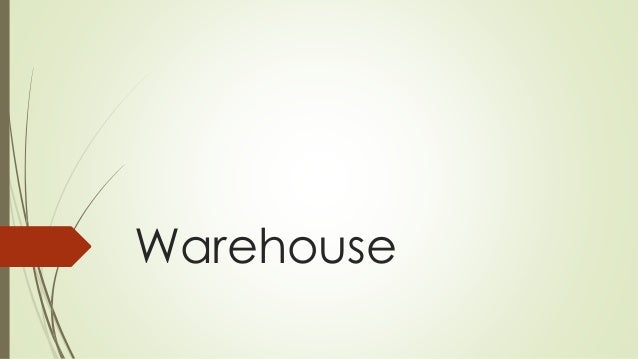The image depicts a minimalistic design with a predominantly light green, almost off-white background, featuring subtle vignetting that makes the edges appear slightly darker. Dominating the bottom left corner is a thin olive green strip that runs vertically from the top to the bottom of the image. Emerging from this strip are several wispy, reed-like lines that curve gracefully, resembling blades of grass. Amidst these lines is a prominent red flag, shaped like a rectangle with a pointed triangle tip, directing attention to the right. Positioned near the bottom left corner, yet somewhat centered, is the single word "Warehouse" in Century Gothic font. The text is black, with only the initial "W" capitalized. An orange or copper-colored arrow originates from the left side, reinforcing the focus on the word "Warehouse." The overall composition suggests a simple, title-slide aesthetic with a natural, slightly aged ambiance.